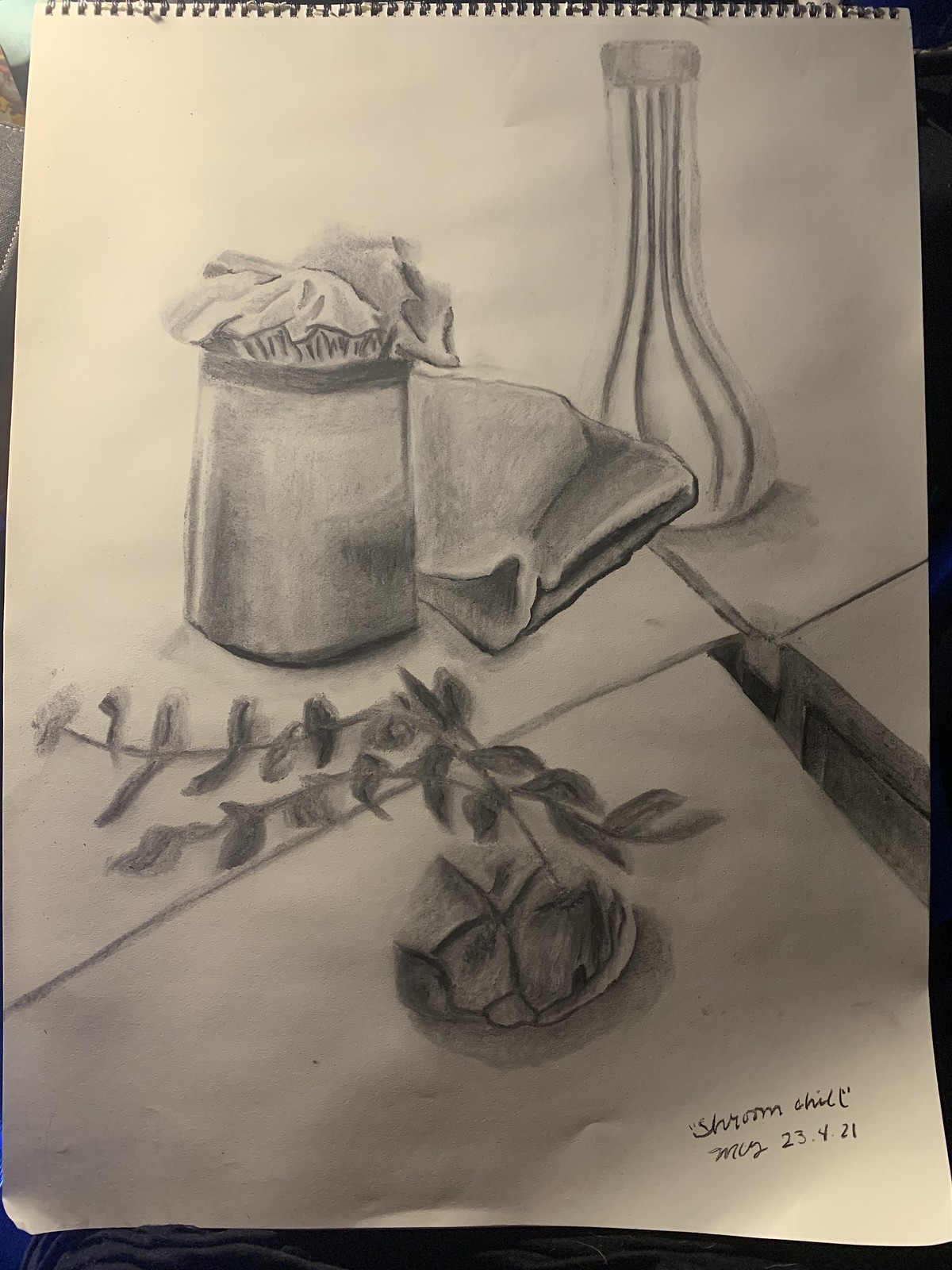A detailed sketch rendered in gray pencil fills the thick white page of a sketchbook. This sketchbook, adorned with tiny metal spirals at the top, takes up most of the image. The paper, though primarily smooth, shows signs of use with slight crumples at the bottom and a few indents. In the bottom right-hand corner, the artist has signed their name and noted the date, marking their creation.

The composition of the sketch is meticulously detailed, featuring an arrangement of various objects. Central to the drawing is a container with pieces of cloth or fabric spilling out, hinting at a soft, textured material. Nearby, a neatly folded piece of cloth adds structure and contrast. A slender, elongated vase stands gracefully beside these items, complemented by delicate sketches of vines or leaves that introduce an element of nature. Positioned somewhat separately, a form resembling a rock adds an organic feel to the assembly. The countertop beneath these objects is also rendered, with a noticeable gap that adds depth and dimension to the scene.